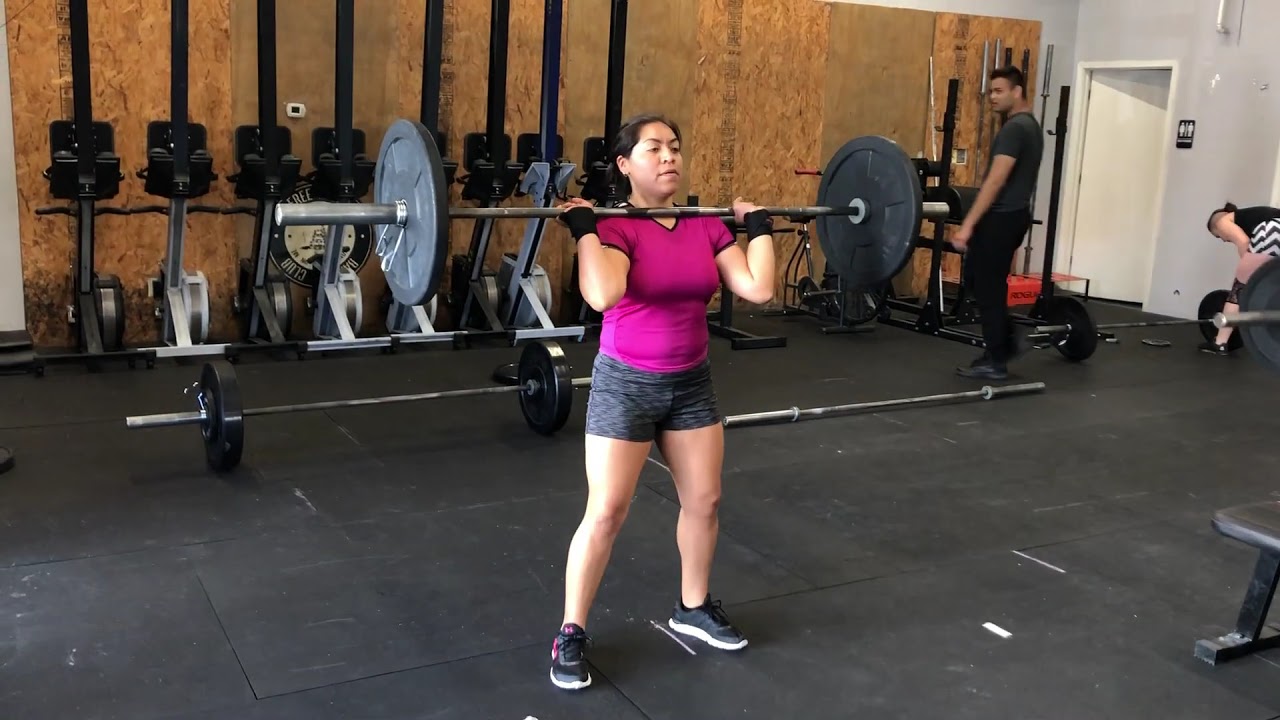In this photograph of a gym, the dark grey floor contrasts with the various exercise equipment scattered throughout the space. The central focus is a woman standing and lifting weights; she wears a pink t-shirt, grey shorts, black shoes with white soles, and appears to be of Filipino or possibly Latina descent. She is holding a large silver barbell with black circular weights on either end. The background features a brown wall with some design elements and an array of black exercise bikes mounted along it. Additional gym equipment and weights are visible behind her. A man and another woman are also present in the gym. To the right, there is a white door likely leading to a bathroom, indicated by a poster beside it. This gym, with its plywood paneling, suggests a more utilitarian and less luxurious setting.